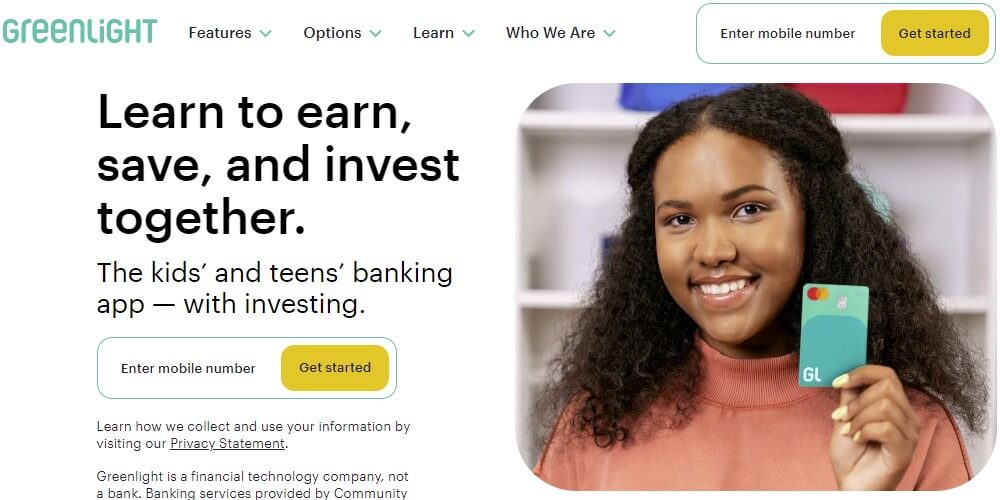This image is a screenshot of the Greenlight website, a banking product designed for children and teens. The Greenlight logo and name are positioned in the upper left corner, stylized in a very light green font with a capital "G" followed by lowercase letters. The top menu includes options labeled "Features," "Options," "Learn," and "Who We Are." 

In the upper right corner, an oblong white box prompts visitors to "Enter mobile number," followed by a gold-colored, rounded-corner rectangle button labeled "Get Started."

The headline on the left side of the page reads, "Learn to earn, save and invest together." Below that, it states, "The kids and teens banking app with investing." A similar prompt for entering a mobile number and a "Get Started" button is also located here.

On the right side, there is a photograph of a young girl, around 12 years old, with medium brown skin and very curly hair that falls just past her shoulders. She is wearing a subtle pink turtleneck and is holding up a Greenlight debit card to the camera. The card is light green and displays the MasterCard logo, characterized by two overlapping circles, one red and one yellow.